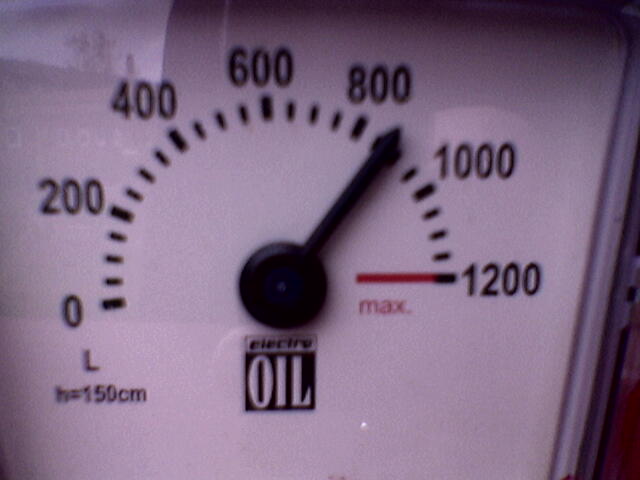This image depicts a detailed view of a mechanical gauge against a white background. The central feature of the gauge is prominently branded with the name "Electro Oil." The gauge appears to measure something on a scale from 0 to 1200, with markings indicating various levels. A red line is visible near the 1200 mark, indicating the maximum level. Below the scale, there is a notation with the letter "L" and the formula "h = 150 cm." 

The gauge needle is positioned between the 800 and 1000 marks, specifically pointing slightly below 900. The background reflects some ambient details, including what might be a tree or a storefront, though these elements are blurry and not clearly readable. The image focuses solely on the gauge, with no other objects present, emphasizing its role in measuring a specific quantity, likely related to oil given the branding.